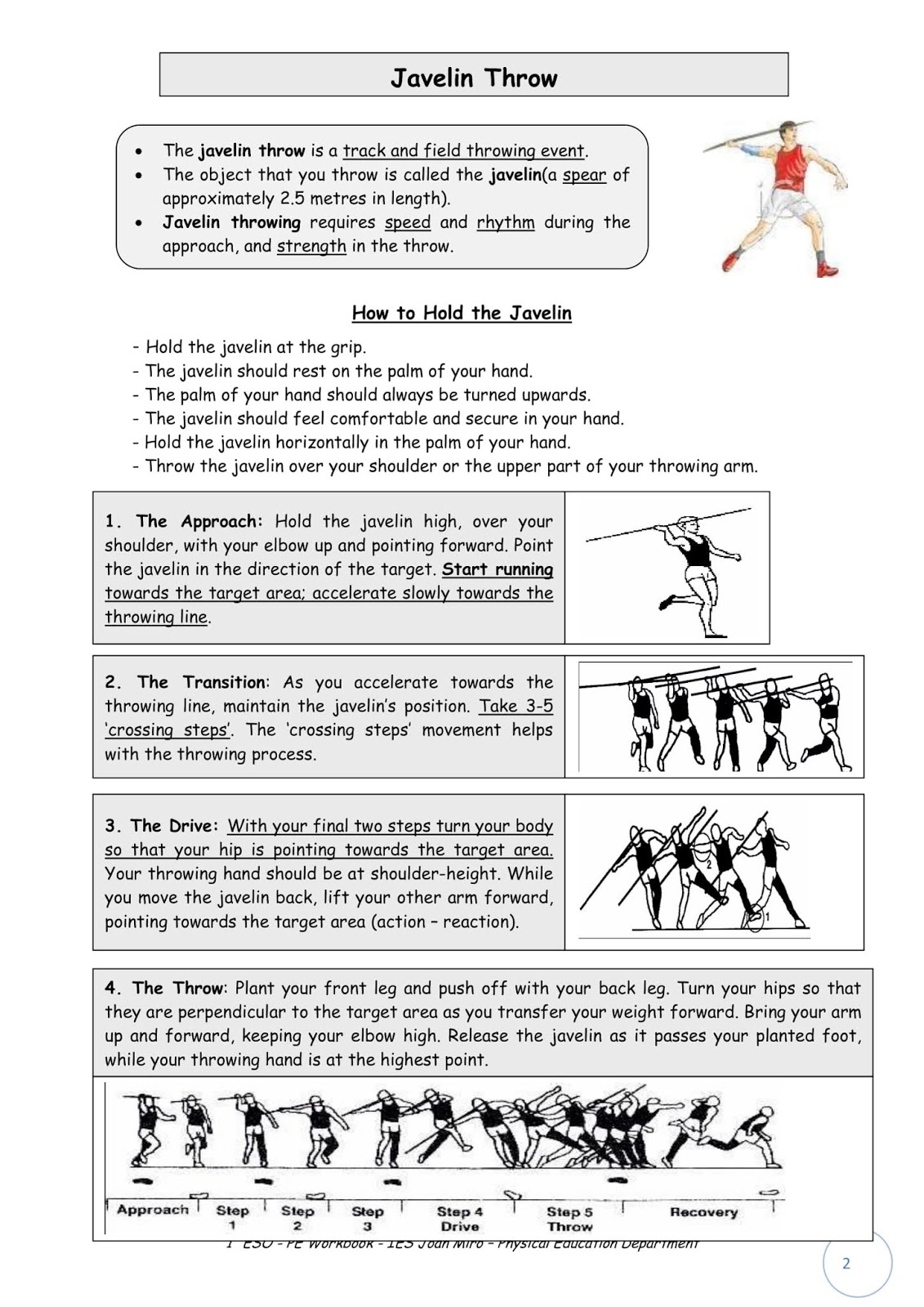The image is an infographic titled "Javelin Throw," providing a detailed step-by-step tutorial on how to throw a javelin. The instruction set, primarily in Comic Sans font, is displayed in basic black and white. On the right side, there is a small colored illustration of a man holding a javelin, ready to throw. The infographic explains that the javelin is a spear approximately 2.5 meters in length, noting the British spelling "metres."

The tutorial is organized into four key steps: 

1. **The Approach**: It illustrates how to hold the javelin high over your shoulder with your elbow pointing forward while running towards the target. Key elements include accelerating gradually and pointing the javelin towards the aim.

2. **The Transition**: Detailed with multiple pen-and-ink line drawings, it describes maintaining the javelin's position while taking three to five crossing steps. This movement is crucial for executing a smooth throw.

3. **The Drive**: The drive step guides you to turn your body so that your hip points towards the target area. You'll lift your throwing hand to shoulder height while using your opposite arm to point toward the target, ensuring the action-reaction principle.

4. **The Throw**: The final step focuses on setting your front leg, pushing off with your back leg, rotating your hips to be perpendicular to the target, and transferring your weight forward. The release of the javelin should occur as the throwing hand reaches its highest point, just past your planted foot.

Each step is supported by black-and-white illustrations that demonstrate the required body postures and movements, providing a comprehensive visual guide from the approach to the recovery phase.